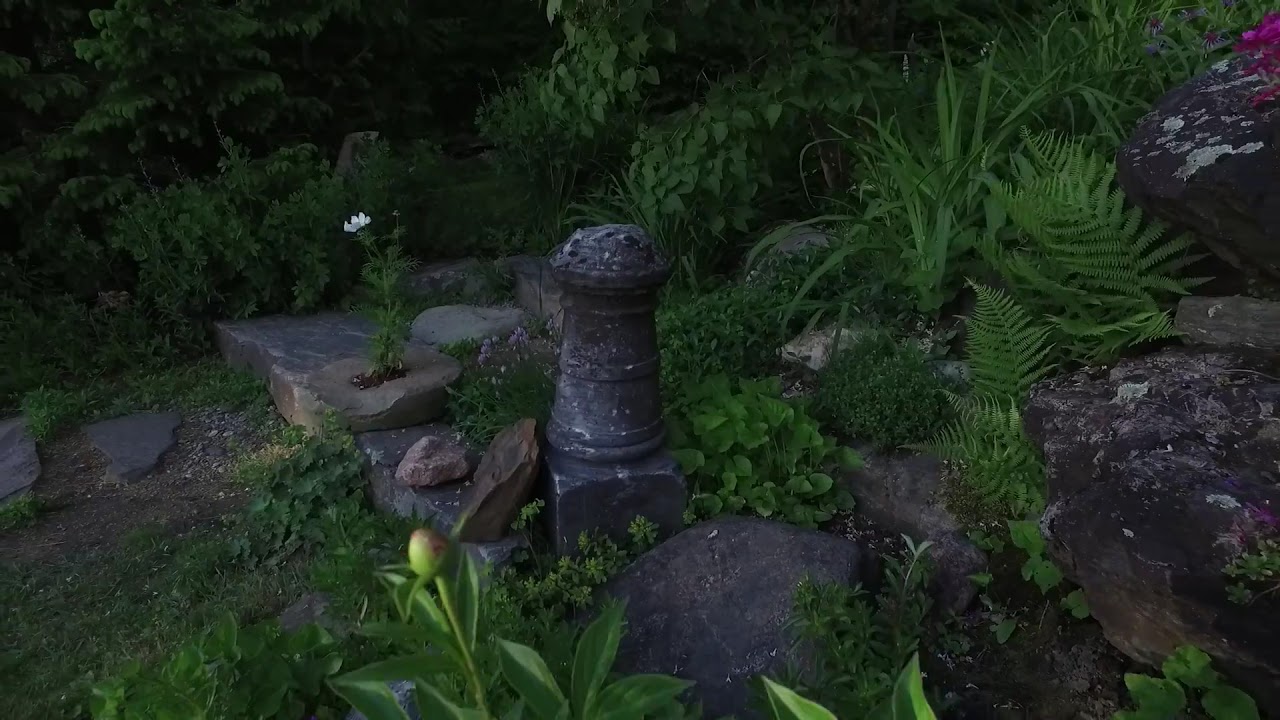The image captures an outdoor rock garden featuring a central stone statue that resembles a chess rook or candle, perched on a pedestal. The statue is primarily dark gray with light black hues. Surrounding the statue are several large, dark gray and black boulders in various shapes, including round and oblong forms. Some of the rocks have cracks, from which small green plants and white flowers emerge. One flower is prominently growing out of a crack in a stone, showing off its stem, leaves, and delicate white petals. Additional budding flowers are visible, poised to bloom amidst the rocks. The scene is enveloped in vibrant greenery, including ferns and fronds that create a lush backdrop. The photograph appears to be taken in low light, suggesting early morning or dusk. In the background, small bushes and trees enhance the verdant ambiance, and there's a hint of a violet flower peeking in from the top right corner. The overall setting is a harmonious blend of rock formations and verdant plant life, creating a serene and balanced natural tableau.